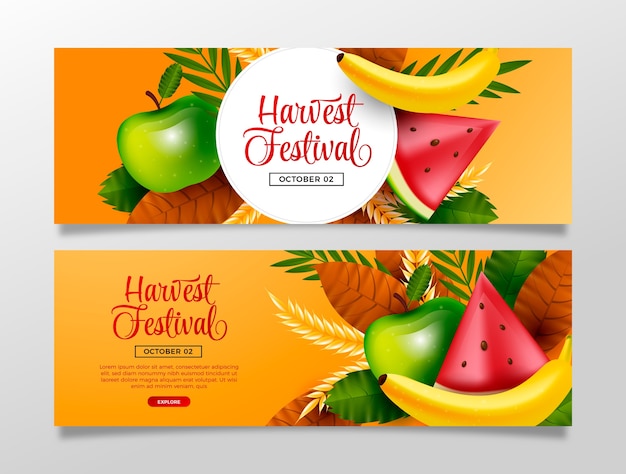The image features a promotional layout set against a light gray background, with two visually striking, orange-hued banners accented by a gradient mixing yellow tones. Both banners are identical in theme and design.

The top banner prominently displays a central white circle containing bold red text that reads "Harvest Festival." Encircling this white circle is a festive assortment of autumnal elements: a yellow banana, a slice of red watermelon, and a collection of vividly colored fruits, including a green apple. These are complemented by a smattering of leaves in shades of green, yellow, and brown, enhancing the seasonal theme.

Below the red text, within a black outlined box, the banner states the event date twice, "October 02, October 02", in black lettering. 

The bottom banner mirrors the design of the top one, featuring the same festive decorations: the yellow banana, the red watermelon slice, a green apple, and a collection of leaves in autumn colors. It also repeats the event details with the red "Harvest Festival" text and "October 02" date.

Both banners cohesively celebrate the Harvest Festival, with their vibrant colors and autumnal imagery promising an engaging and festive event.